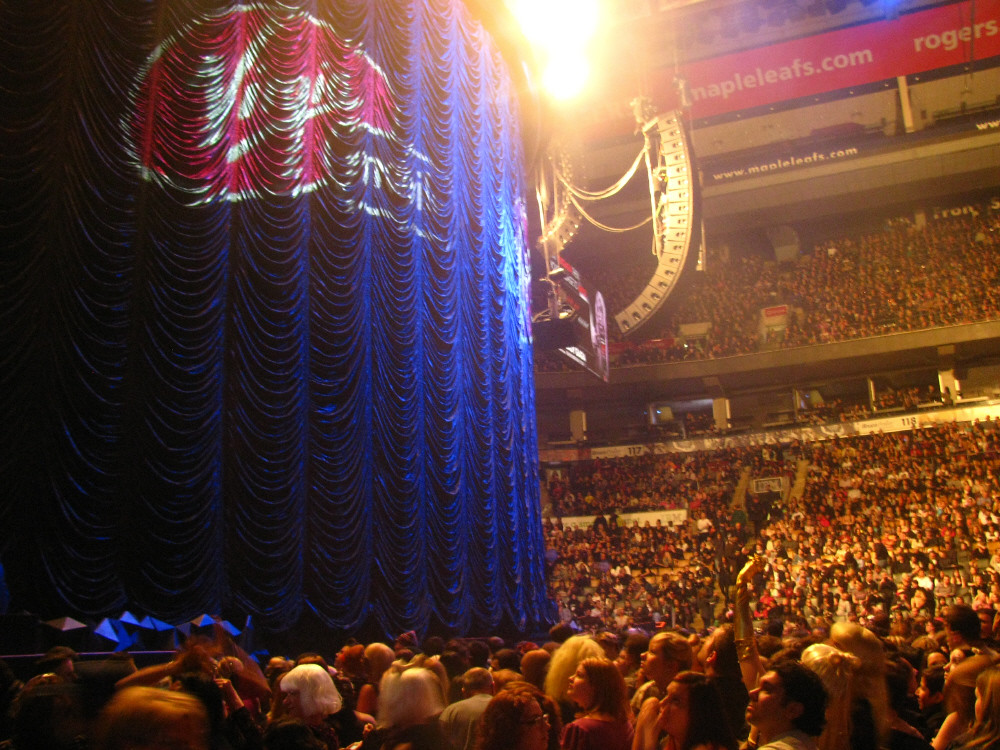The picture depicts an expansive, packed stadium during what appears to be a rock concert or similar event. The central focus is a massive blue curtain occupying about a third of the left side of the image, illuminated by a golden light. This curtain prominently features the Virgin logo in a red balloon, indicating sponsorship by Virgin Mobile. The crowd, numbering in the thousands, fills every seat from the front rows to the upper grandstands and balconies, extending all the way to the rafters. Advertisements and signs, including those for mapleleafs.com and Rogers, are scattered around the gray stone stadium. The arena is rounded, suggesting a central stage hidden behind the curtain, and a bright light emanates from the ceiling, enhancing the overall atmosphere of anticipation among the audience.